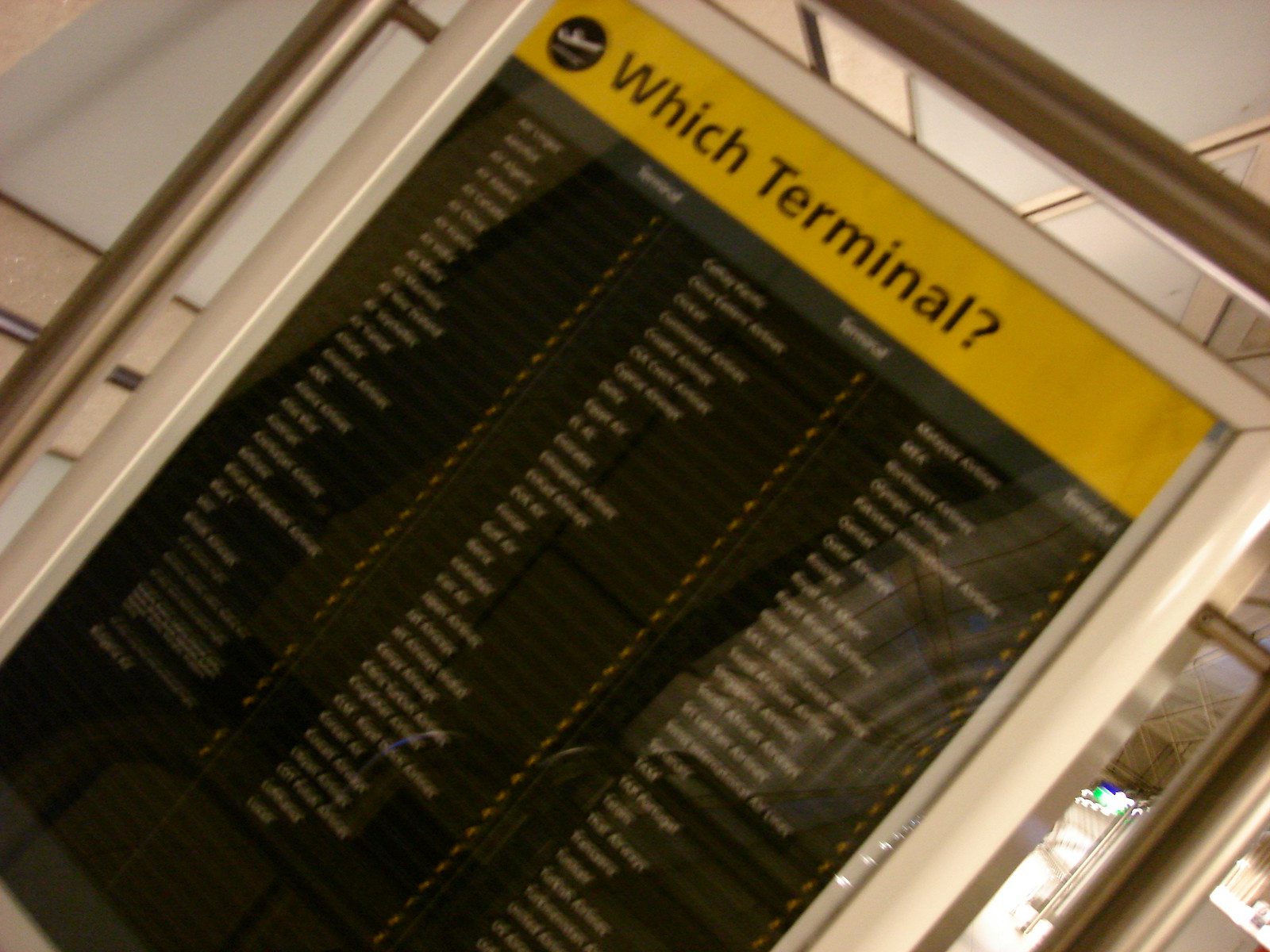This photograph, taken inside an airport, captures a large informational sign titled "Which Terminal?" situated prominently in the center. The image is angled at approximately 45 degrees, suggesting it was quickly taken using a smartphone. The sign is framed in silver with yellow and black detailing. At the top is a yellow banner featuring a black circle with a white outline of an airplane taking off, alongside the text "Which Terminal?" in black. The main body of the sign has a dark background with three columns of white text presumed to be destinations, indicated by the layout and design. Although the text is too blurry to read clearly, each destination is followed by a number and marked with yellow accents. The surrounding environment includes elements of the airport's architectural features, with white and gray or tan walls and a blue line visible on the top left. The overall snapshot, while blurrier and tilted, encapsulates the essential information and bustling atmosphere of the airport setting.